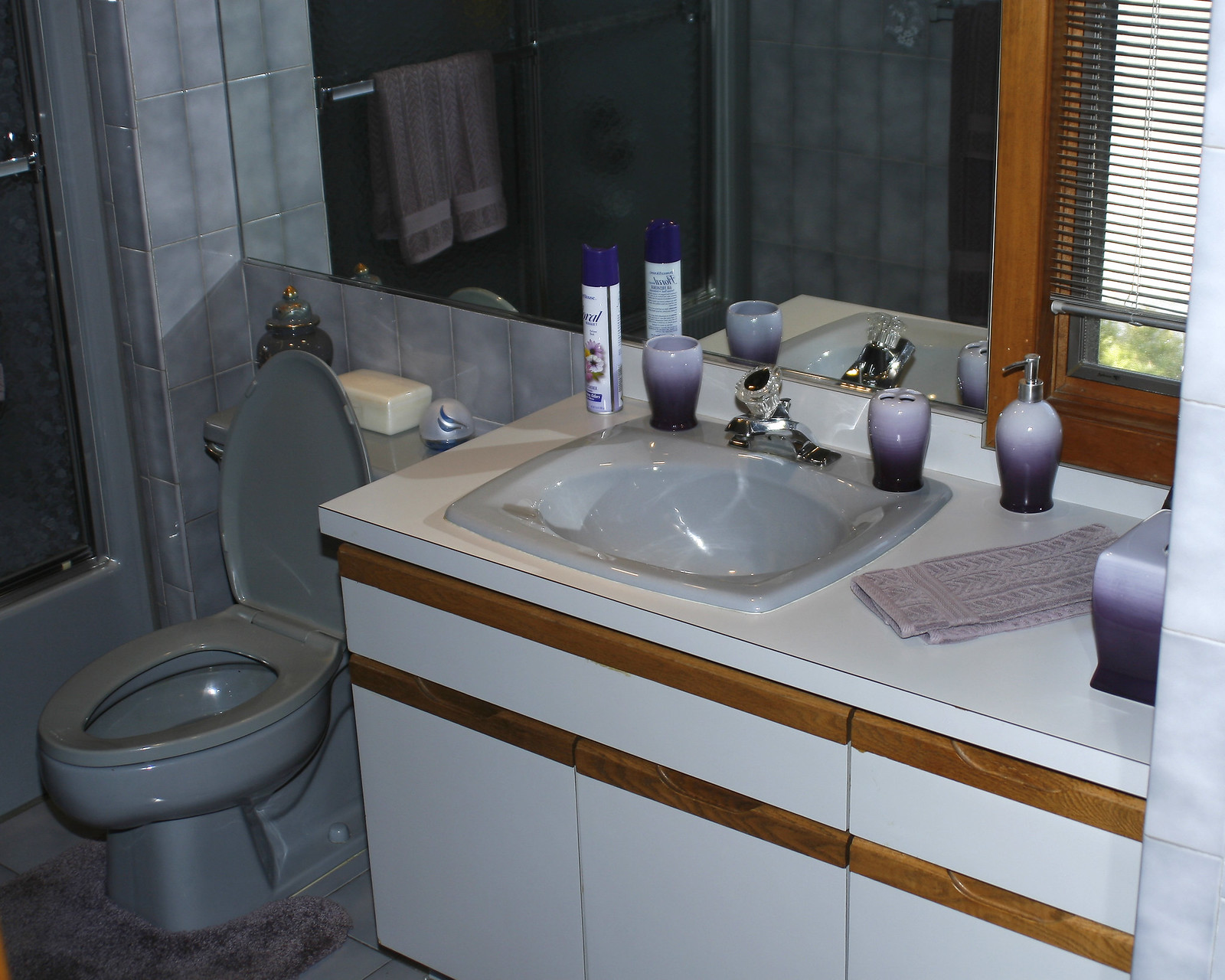The image depicts a bathroom with a distinctly 1990s aesthetic, characterized by its primarily white color scheme and tiled walls. The room features a unified porcelain finish across the sink, toilet, and tub shower. The sink area includes a white wooden vanity with wood trim edges, topped with a white counter that houses the inset porcelain sink, which is equipped with a silver spout.

Touches of purple are evident throughout the bathroom, adding subtle accents to the otherwise neutral palette. These purple elements include a toothbrush holder, lotion or soap pump, a cup, a toothbrush holder, a tissue dispenser, a hand towel, and an air freshener. The color of the tiles also hints at a purple undertone, blending seamlessly with the other accents.

Positioned behind the toilet, there is a small white holder for wet wipes and an air purifier or air freshener. The bathroom features a wooden-framed window adorned with blinds that are drawn up to allow natural light to enter.